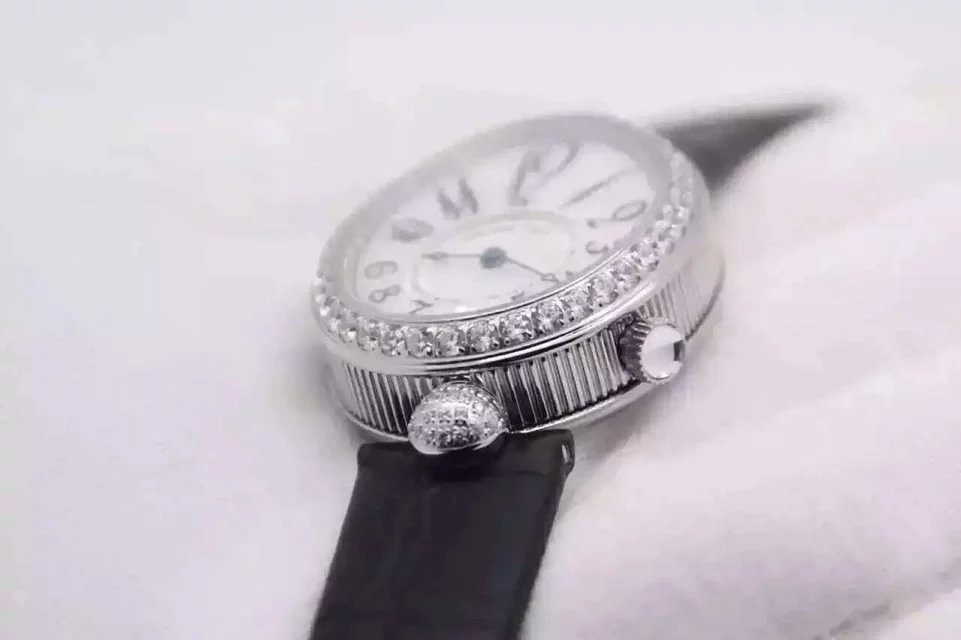In this detailed black and white photograph, we are presented with an exquisitely crafted wristwatch set against a pristine white background. The watch features a sophisticated black band, paired with a luxurious white gold or silver casing, whose true color is indistinguishable in the monochromatic image. The upper edge of the watch face is elegantly adorned with a row of small diamond chips, counting approximately 30 to 40, adding a touch of glamour and refinement. At the 3 o'clock position, there is a small wind-up crown. The watch face sports a clean, white background with bold black numerals and sleek black hour and minute hands, silently indicating the time as 9:20. The absence of a second hand highlights the minimalist yet opulent design of this timepiece, making it a striking combination of functionality and elegance.